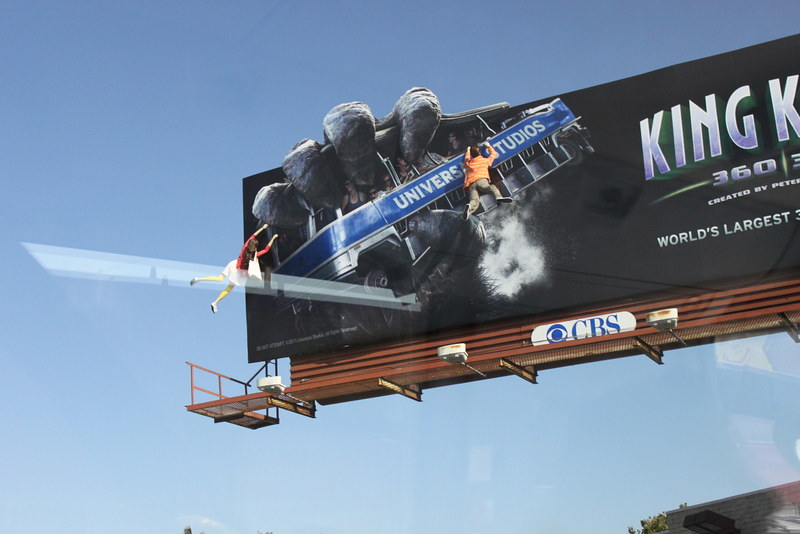This photograph captures a striking, close-up view of a billboard set against a clear blue sky. The billboard itself, only partially visible, features a predominantly black background. On the right side, although truncated, it displays the text: "King K 360, created by Peter, world's largest." Dominating the left side of the image is a dramatic 3D element: an enormous black hand gripping a trolley cart designed to resemble a bus labeled "Universal Studios." Adding to the dynamic scene, two realistic mannequins are seen hanging off the bus, appearing as though they have been thrown out. This visually compelling billboard is an advertisement for a King Kong ride or experience, part of the Universal Studios theme park's backlot tour.